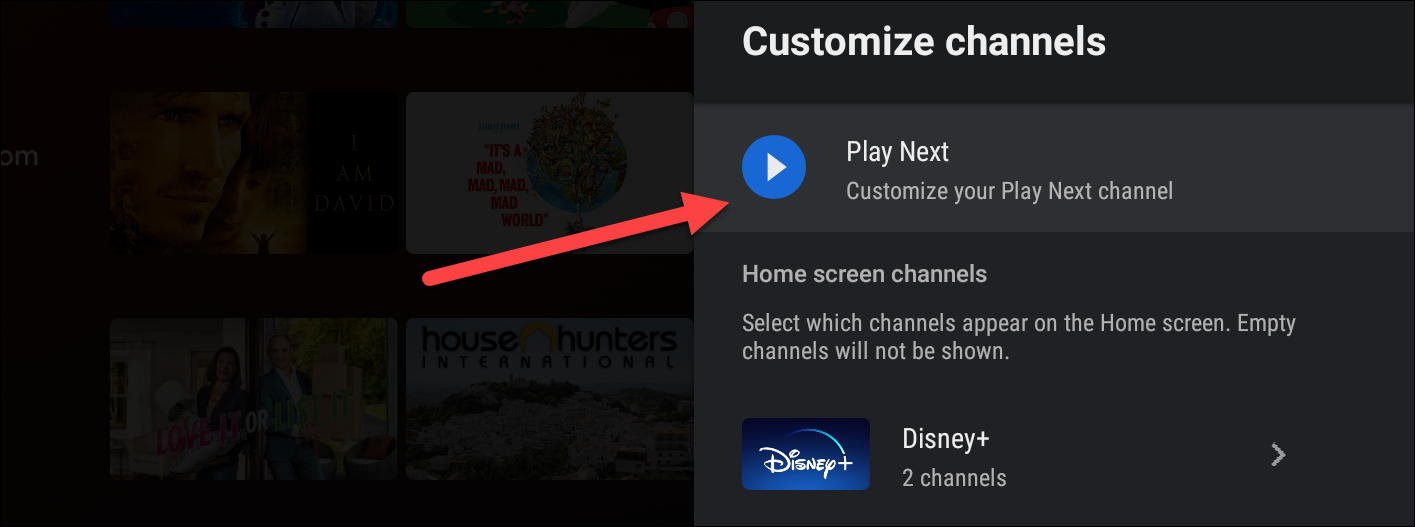The image consists of several layered elements with varying degrees of visibility. Dominating the right side of the foreground is a prominent textual overlay that reads "Customize Channels" in bold, white text. Below this heading is a blue button labeled "Customize Your Play Next Channel,” highlighted by a red arrow to draw user attention, suggesting an interactive cue to click or focus on it.

Directly beneath the blue button, there is a section titled "Home Screen Channels" accompanied by instructional text explaining, "Select which channels appear on the home screen. Empty channels will not be shown." Adjacent to this instruction is a small Disney Plus icon, indicating that two channels under it are currently selected or available.

In the background, there is a faint, semi-transparent arrangement of show or program icons, the most discernible being "House Hunters International." These background elements provide a subtle context without overshadowing the primary focus.

Overall, the image's intent is clearly to guide users on how to customize their viewing experience, specifically emphasizing the "Play Next" feature by indicating where and how to interact with it. The design is clean, with the critical interactive elements prominently displayed for ease of navigation and user engagement.